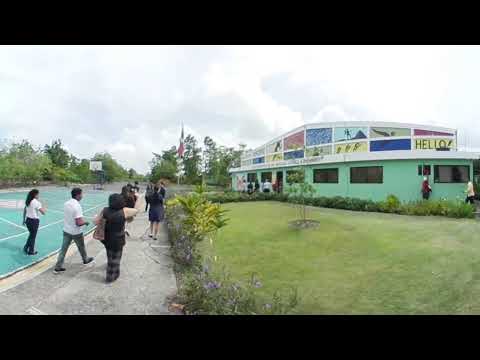In this vibrant image, a group of people are walking down a cement sidewalk that runs along the left side of the frame. On the left edge of the sidewalk, there's a green basketball court with white lines and a visible hoop. One woman in the group is wearing a white shirt and black pants and appears to be walking on the court itself. To the right of the sidewalk is a well-manicured lawn featuring a single small tree at its center. The lawn is bordered by a variety of plants and a hedgerow. 

Further right and beyond the hedgerow, stands a tall, brightly-colored turquoise building with a distinctive domed roof. The dome is decorated with colorful rectangular panels, each containing different pictures. There is a gathering of people near the entrance of this eye-catching building. The scene is set under a clear sky with fluffy clouds, signifying a bright and pleasant day. Toward the distance, there's a flag visible, though its details are not clear. Black horizontal lines frame the top and bottom of the image, giving it a structured feel.